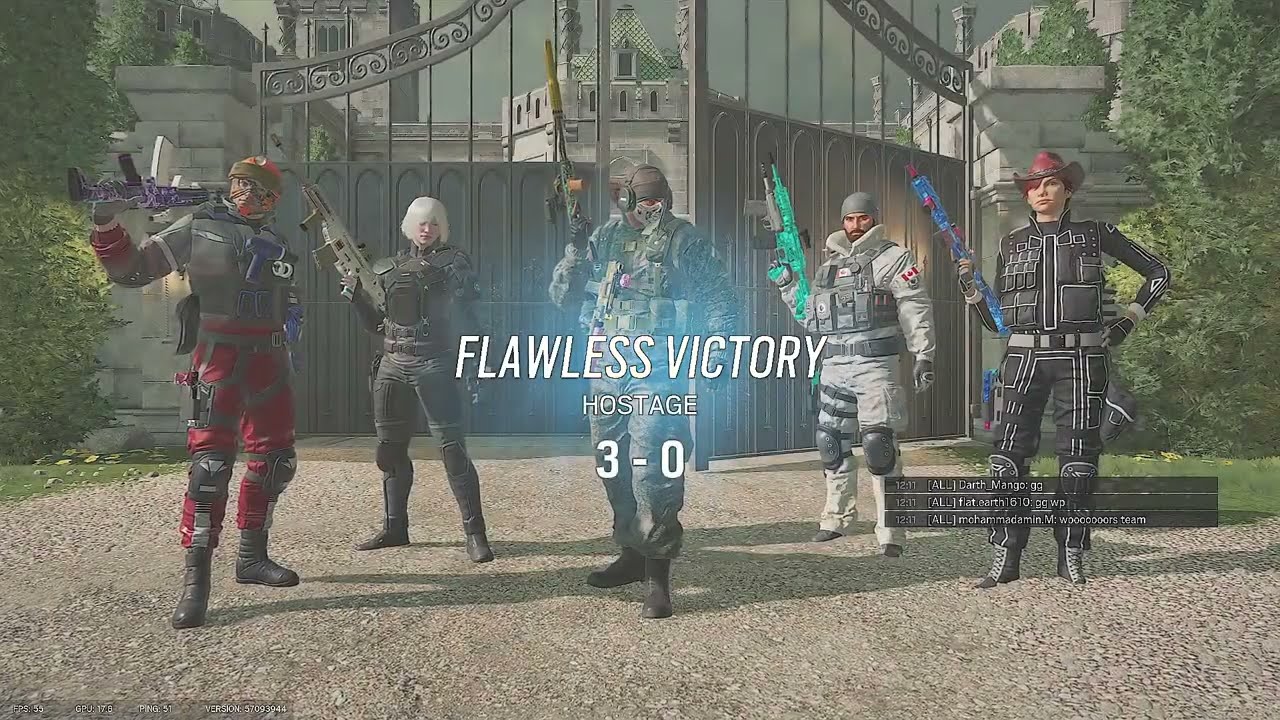In this image, we see a detailed screenshot from a video game. The background features an unpaved road and a partially opened wrought iron gate with concrete pillars on either side, situated among trees and bushes. The scene is dominated by five video game characters, standing in a line directly in the center of the image, all holding guns and staring darkly at the camera. The text "Flawless Victory Hostage 3-0" is prominently displayed in the center.

Beginning with the character on the far left, he stands out with an orange helmet concealing his face, a green vest, red pants, and is holding a rifle over his shoulder. Next to him, the second character has white hair and is dressed in an all-black uniform. The central character, donning a helmet and headphones, is outfitted in camouflage and is aiming a rifle. To his right, the fourth character is prepared for cold weather, wearing a snowsuit with knee-pads and three black bands on his right leg, and carrying a translucent neon green gun. He also features either a toboggan or a do-rag. Finally, on the far right, the last character wears a black-and-white outfit including a gray belt, a distinct red cowboy hat, and a blue gun, with red hair falling onto his forehead.

The color palette comprised in the image includes shades of gray, green, red, light blue, blue, tan, silver, and additional hues of green. The entire composition, with its diverse characters and detailed setting, clearly illustrates a dramatic moment from the game's storyline.